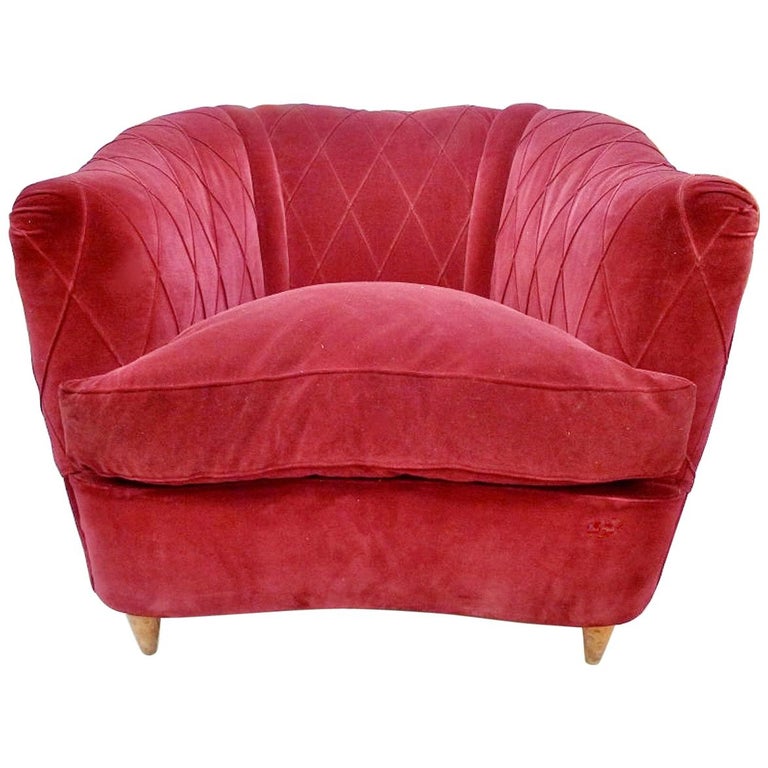This is an image of a large, overstuffed armchair upholstered in plush burgundy velvet. The chair features a distinctive curved back and seat, both of which are exceptionally padded, giving it a fluffy, inviting appearance. The backrest is quilted with an interlocking diamond pattern, adding an elegant touch to the design. The two front legs are short, cone-shaped, and made of wood, providing sturdy support. The armchair's seat cushion is slightly raised and curved, making it spacious enough to comfortably accommodate two smaller individuals. The upholstery, while still rich in color and texture, shows signs of use without any noticeable defects. The background of the image has been edited out, suggesting that this is a product image intended for sale.